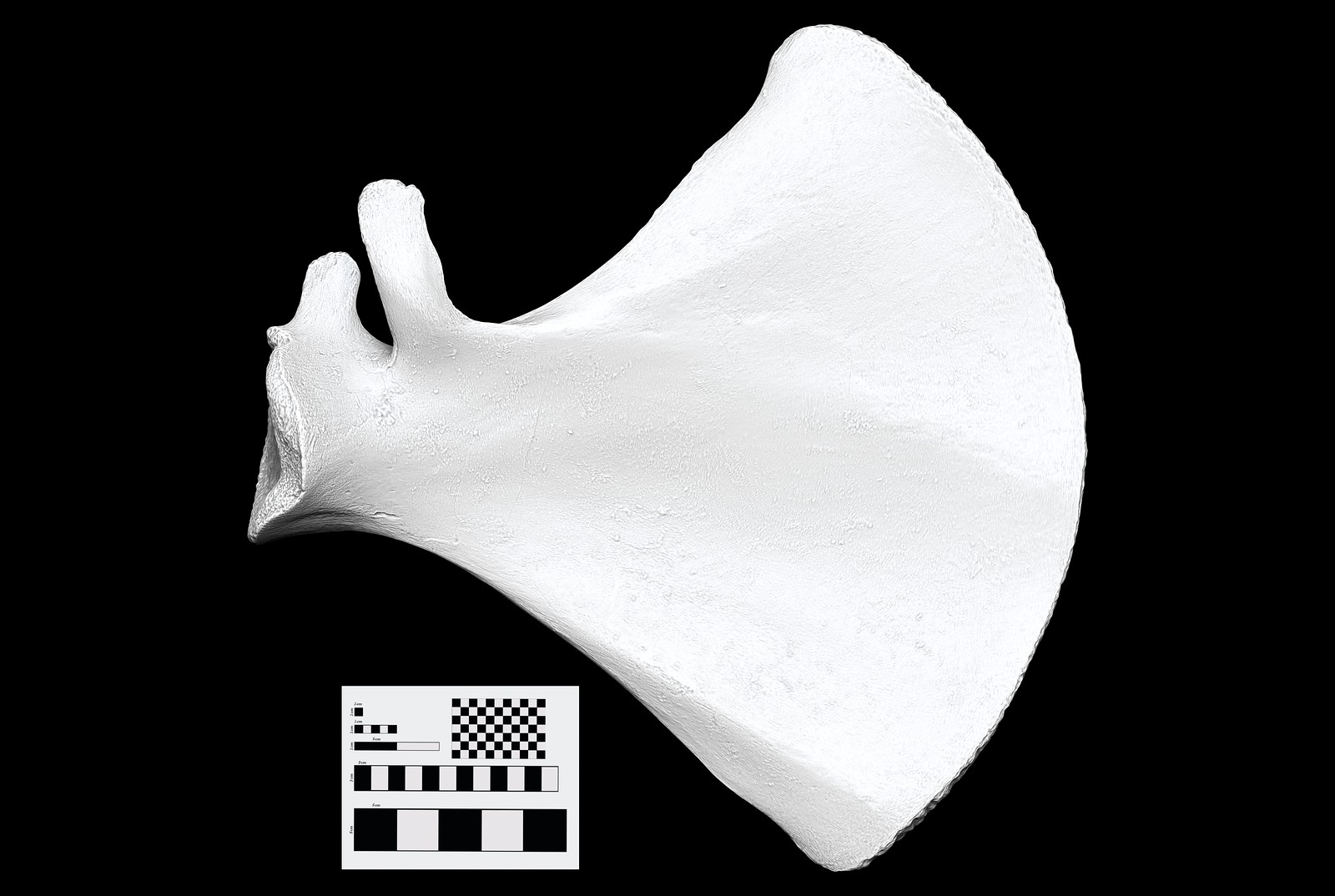The image features an all-black background with a striking white object at its center, which resembles a curved shape that could be interpreted as a broken-off bone, a shoulder blade, or even a seashell. This central white object curves into a large half-circle on the right and tapers leftward into a triangular form with two notches on the upper left side. Below this object, a smaller white rectangle contains a variety of black and white patterns. At the top of this rectangle, there is a checkerboard pattern of black and white squares. Below the checkerboard, there are sequential black and white squares and lines, including alternating black and white rectangles, and a final row of five alternating black and white squares at the bottom. This is the only color contrast within the image, emphasizing the stark distinction between black and white elements.